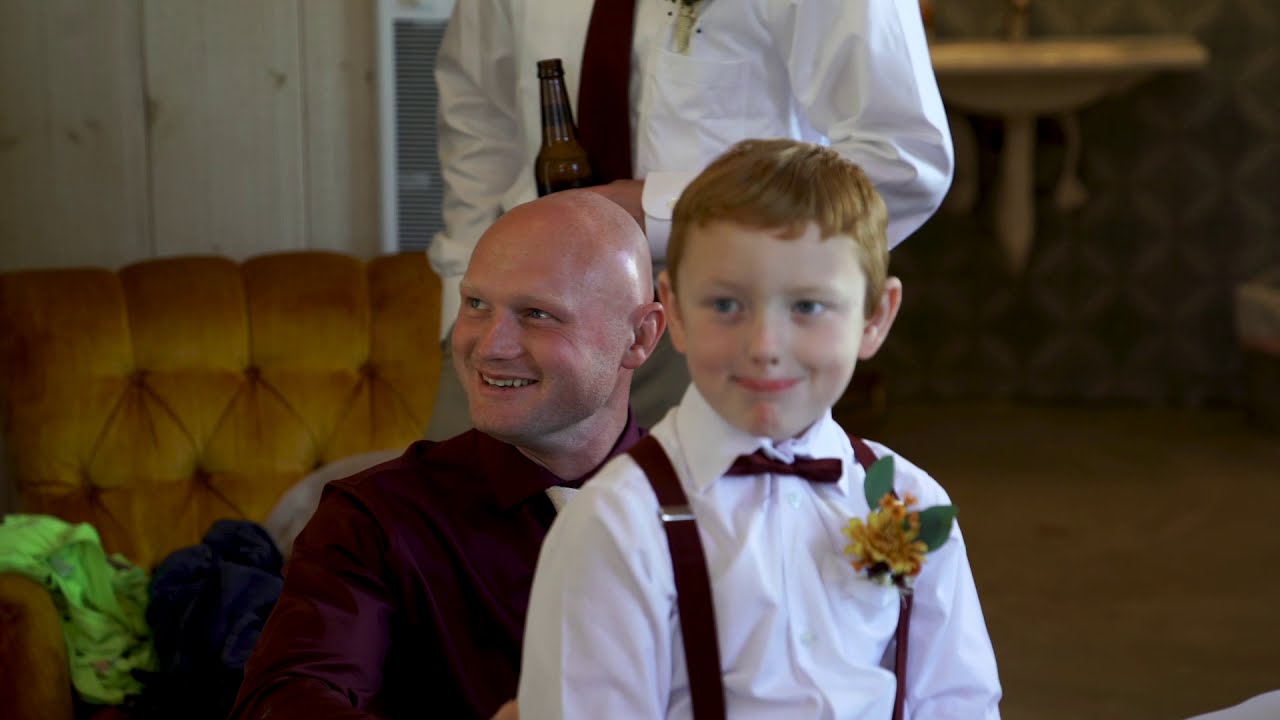In this detailed photograph, a joyful little boy, around eight years old, with short red hair and a cheerful grin, sits on a bald man's lap. The boy is elegantly dressed in a white long-sleeved button-up shirt, dark red bow tie, and matching suspenders. A yellow flower with green leaves adorns his pocket. He gazes slightly to his left, adding a charming touch to his appearance. 

The man holding him has turned his head to the left, smiling so widely that his teeth are visible. He, too, is dressed formally in a dark jacket and tie, and appears to be enjoying the moment, indicated by his broad smile. His blue eyes and bald head are prominent features. 

Standing behind them is another man, visible from about the shoulders down. This man is wearing a white shirt with a black tie and has a flower pinned on his left chest, similar to the boy. He holds a brown beer bottle in one hand. The background includes a light green shirt draped over the armrest of a recliner and a plush yellowish couch or chair, possibly velvet, with a wooden wall and a white vent or furnace against it, suggesting the cozy setting of a post-wedding celebration.